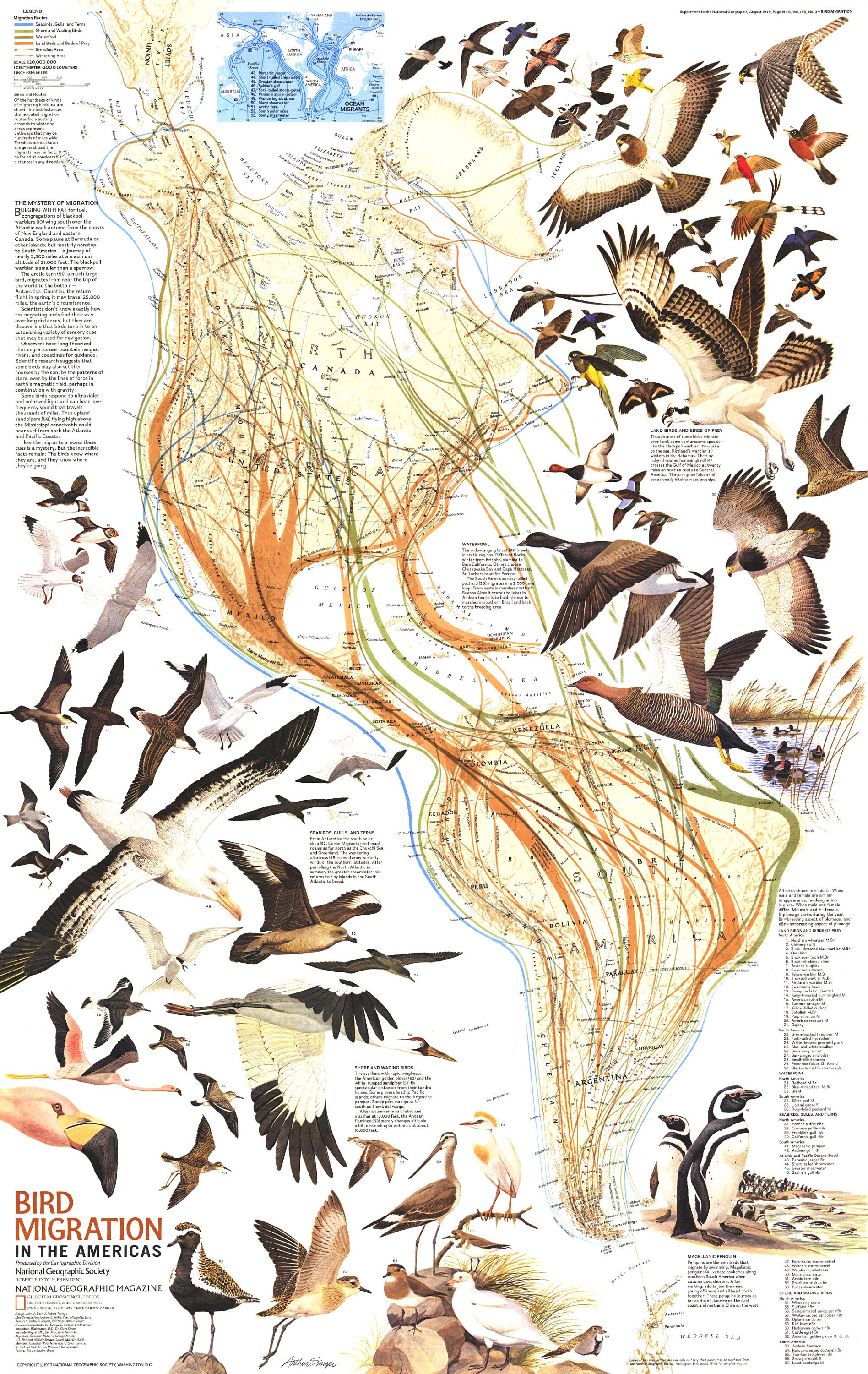This detailed image from what appears to be a National Geographic magazine or textbook page presents a comprehensive map that spans North America, Middle America, and South America, illustrating the migration paths of various bird species. The map, predominantly light yellow, features a network of orange, green, and yellow lines depicting the diverse migratory routes. Accompanying this map are numerous illustrations of birds, encompassing a broad spectrum from hawks to penguins. Scattered across the image are multiple paragraphs of text detailing the flight paths and behaviors of these birds, including labels such as land birds, birds of prey, waterfowl, and ocean migrants. The top left corner hosts a legend for interpreting the map, as well as a long paragraph that delves into the mystery of bird migration. The image is captioned "Bird Migration in the Americas" in the bottom left corner, underscoring the National Geographic Society's dedication to illuminating this natural phenomenon.